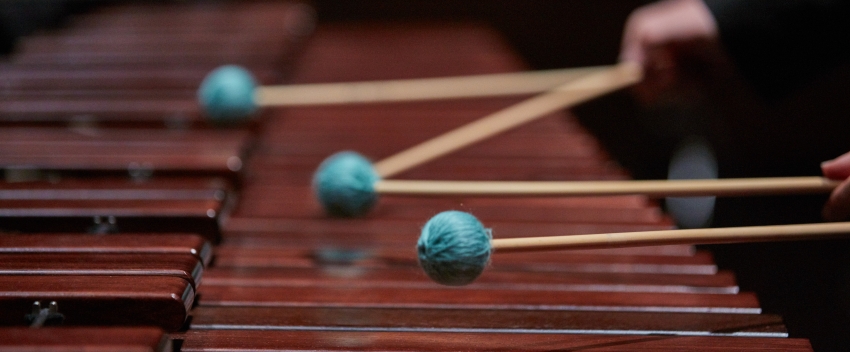This image captures a detailed view of a large, wooden xylophone with a pronounced woodgrain brown color. The xylophone consists of two layers of keys, with one layer slightly stacked atop the other. In the image, two blurred hands are visible, each holding a pair of mallets. The mallets feature light wooden handles, possibly bamboo, with tips made of blue-green yarn, resembling balls of yarn. The hands are positioned over the xylophone, indicating that the individuals are in the process of playing the instrument, with the mallets poised to strike the keys.